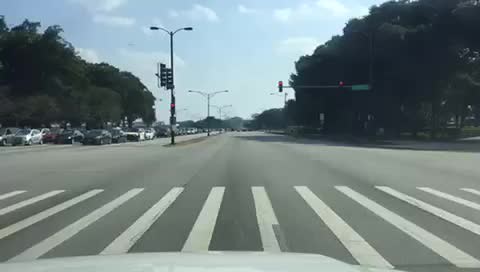A driver's-eye view from inside a vehicle stopped at a red light shows a crosswalk in front and a clear lane extending straight ahead. Large, lush green trees frame the scene on both the left and right sides. The driver is at the front of the line, with no vehicles ahead. The sky is a brilliant blue dotted with a few clouds, indicating a bright daytime setting. To the left, the opposite lane is filled with numerous cars waiting at their own red light. Streetlights positioned in the median cast their glow over both lanes, adding a subtle urban touch to the verdant surroundings.